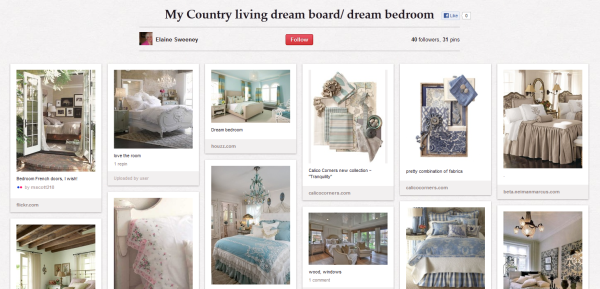This screenshot showcases a Pinterest board titled "My Country Dream Board/Dream Bedroom" by user Elaine Sweeney. Her profile picture is displayed alongside a red "Follow" button, indicating her presence on the platform. Elaine's profile boasts 40 followers and 31 pins, emphasizing her engagement within the Pinterest community. 

The board itself features approximately 12 pins, predominantly focusing on bedroom aesthetics with a few dedicated to living room decor. The overall theme gravitates towards cozy, country-inspired interiors with a casual and comfortable vibe. The decor is highlighted by pastel hues and predominantly showcases various bed sheet arrangements and how the beds are styled. 

One standout pin displays a charming bedroom with French doors adorned with flowers, creating an inviting and serene atmosphere. Another pin features a bedroom exuding English countryside elegance, complete with a chandelier, large windows, and two mounted paintings that enhance its rustic charm.